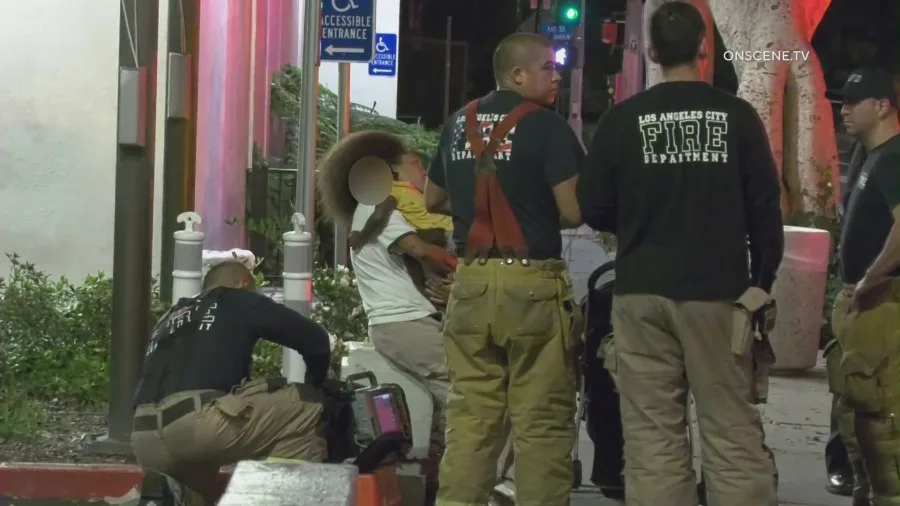The nighttime outdoor photo features a small courtyard scene involving several members of the Los Angeles Fire Department. The firefighters, dressed in long-sleeve black shirts with "Los Angeles Fire Department" inscribed in white—some letters styled with the American flag—are seen engaging in an emergency response. They wear standard tan firefighter pants, creating a uniform yet slightly casual appearance. One firefighter kneels on the left, while others stand nearby. A woman in a white shirt and chino pants, her face blurred, sits on a bench holding an Afro-haired baby. Nearby signage, including multiple indications of handicap-accessible entrances, adds context to the location. Streetlights and a large tree frame the background, revealing a dark sky, and the logo "onscene.tv" appears prominently in the upper right corner of the image.